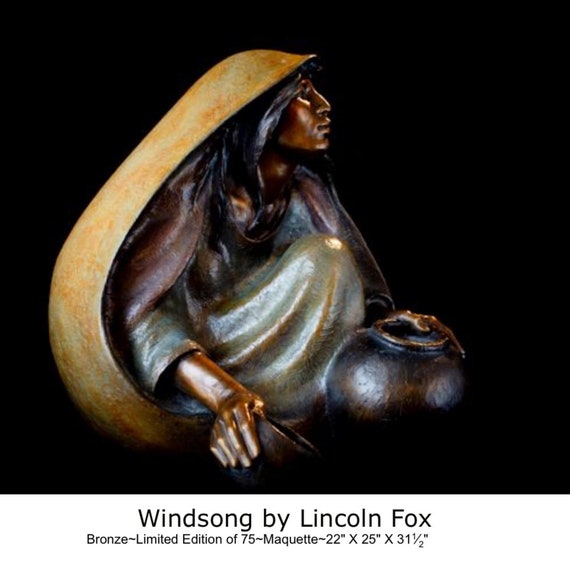This detailed photograph captures a vibrant bronze sculpture titled "Wind Song" by Lincoln Fox, set against a pitch-black background that accentuates the intricate details and painted elements of the artwork. The sculpture, part of a limited edition of 75 maquettes, standing at 22 by 25 by 31.5 inches, depicts a crouched indigenous woman with long black hair, her bronze-colored skin and features gleaming under the lighting. She is adorned in a maroonish cloak and a greenish-gray dress, with a distinctive, yellowish gold, smooth hood that elegantly curves from her head around the left side of her body, reminiscent of a veil or mantle. In her left hand, she holds a vase, while her right hand clutches a bowl, suggesting the act of scooping water. Her expression is one of contemplation, adding depth and a profound sense of narrative to this beautifully crafted piece. Below the image, the text reads: "Wind Song by Lincoln Fox. Bronze, limited edition of 75, maquette, 22 by 25 by 31 and a half inches."